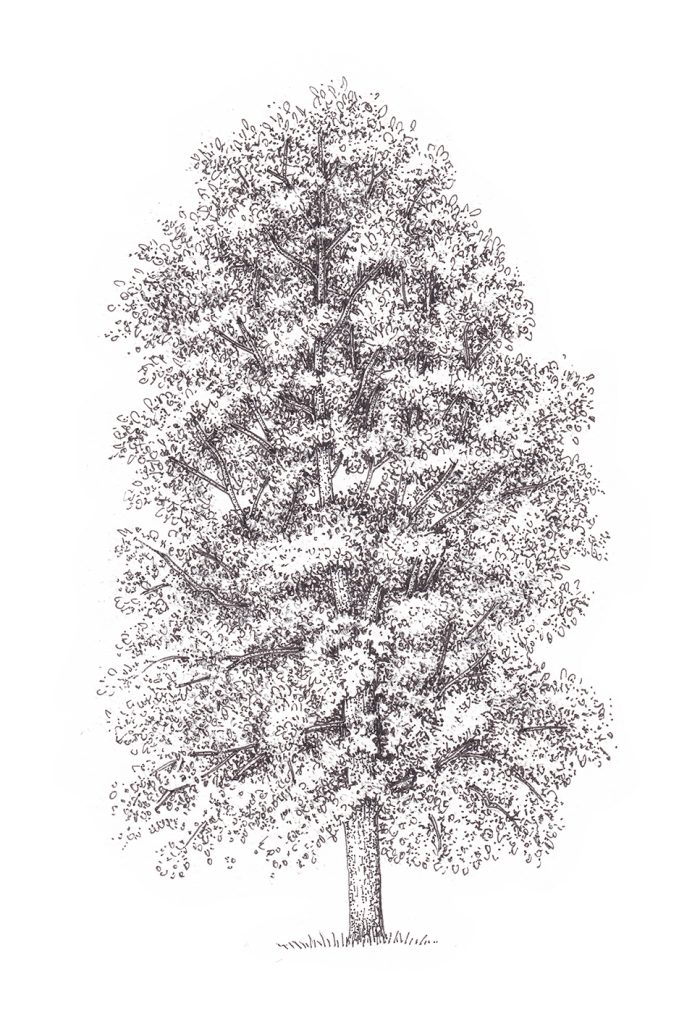This black and white drawing presents a very tall and oblong-shaped tree, likely an oak, in full bloom. The simple yet detailed pencil sketch showcases the tree set against a white background, with a narrow trunk that extends all the way up, visible through the densely packed branches and leaves. The base of the tree features a tuft of grass, adding a touch of realism to the scene. The branches are nearly full to the ground, giving the tree a heavy and robust appearance, indicative of summertime. Despite its simplicity and lack of color, this highly detailed sketch resembles a botanical illustration or a diagram, possibly intended for educational purposes or as a coloring page. The careful rendering suggests it could be used to identify this type of tree, blending seamlessly with the blank background.